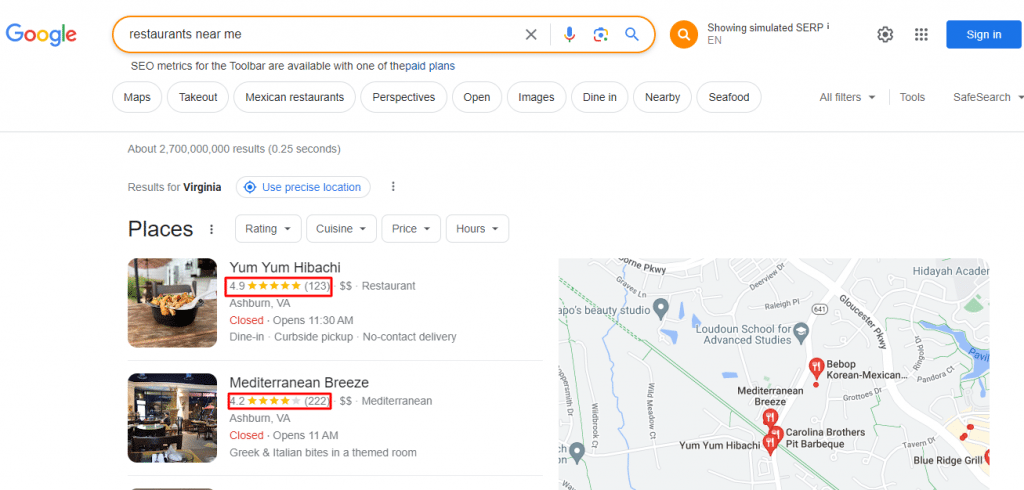**Caption:**

In this detailed close-up screenshot, a user has performed a Google search for "restaurants near me." The familiar Google logo is positioned in the top left-hand corner, with the search bar located to its right. Within the search bar, icons for stopping voice input, searching by photo, and manually typing input, as well as an additional search icon with an orange background, are visible. Beside them are typical icons such as the settings gear, a clickable menu, and the blue sign-in button.

Beneath the search bar, a message mentions the availability of SEO metrics for paid plans. The user interface includes tabs for Maps and Takeout, and below these, various filters such as "Mexican," "Open Now," "Images," "Dine-In," "Nearby," and "Seafood" are offered. Additional options like "Tools" and "SafeSearch" are also provided. The search has yielded approximately 2.7 billion results in 0.025 seconds, specifying the location as Virginia and suggesting the use of precise location for more accurate results.

Among the search results, the first listing is for "Yum Yum Hibachi." This restaurant boasts a 4.9-star rating from 123 reviews, has a price range indicated by two dollar signs, and is located in Ashburn, Virginia. Although currently closed, it will reopen at 11:30 a.m., offering dine-in, curbside pickup, and no-contact delivery services. An accompanying image displays a bowl of Hibachi food on a brown table.

Following Yum Yum Hibachi, the next result is "Mediterranean Breeze," rated 4.2 stars from 222 reviews. It is also marked by two dollar signs, indicating affordability. Located in Ashburn, Virginia, this restaurant will reopen at 11 a.m., offering Greek and Italian dishes in a themed dining room. A photo to the left shows the restaurant's interior, complete with windows and tables.

To the right of these results is a small map highlighting the locations of several restaurants, including Bebop Korean Mexican, Mediterranean Breeze, Carolina Brothers Pit Barbecue, and Yum Yum Hibachi. The Blue Ridge Grill is marked farther east, nearly off the map. The map provides a visual summary pinpointing each restaurant in Ashburn, Virginia, where the user is currently searching for dining options.